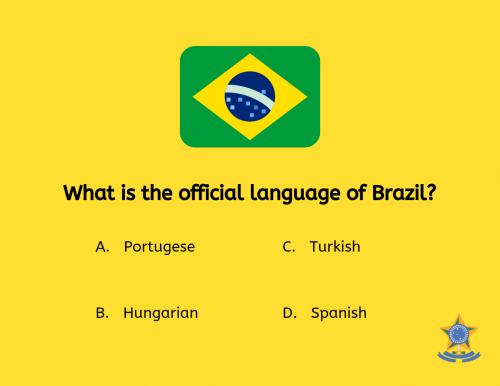This image is a colorful and intricate visual, likely from a language quiz or educational resource. The background is a yellow square. At the center of this square is a smaller green box, which itself contains a yellow triangle. Inside the triangle, there is a small round blue circle adorned with dots and a line in varying shades of blue. 

Below this central motif, a quiz question is written in black lettering: "What is the official language of Brazil?" Directly beneath the question are four multiple-choice options, each also in black text:

- A. Portuguese
- B. Hungarian
- C. Turkish
- D. Spanish

In the bottom right-hand corner of the image, there is a five-pointed star outlined in yellow, with each point colored blue. The center of the star is circular and blue, featuring small white dots. Extending from the bottom of the star is a white line, with blue lines curved beneath it in a manner resembling a rocking chair. The overall design suggests that this page is from a quiz or language learning material.